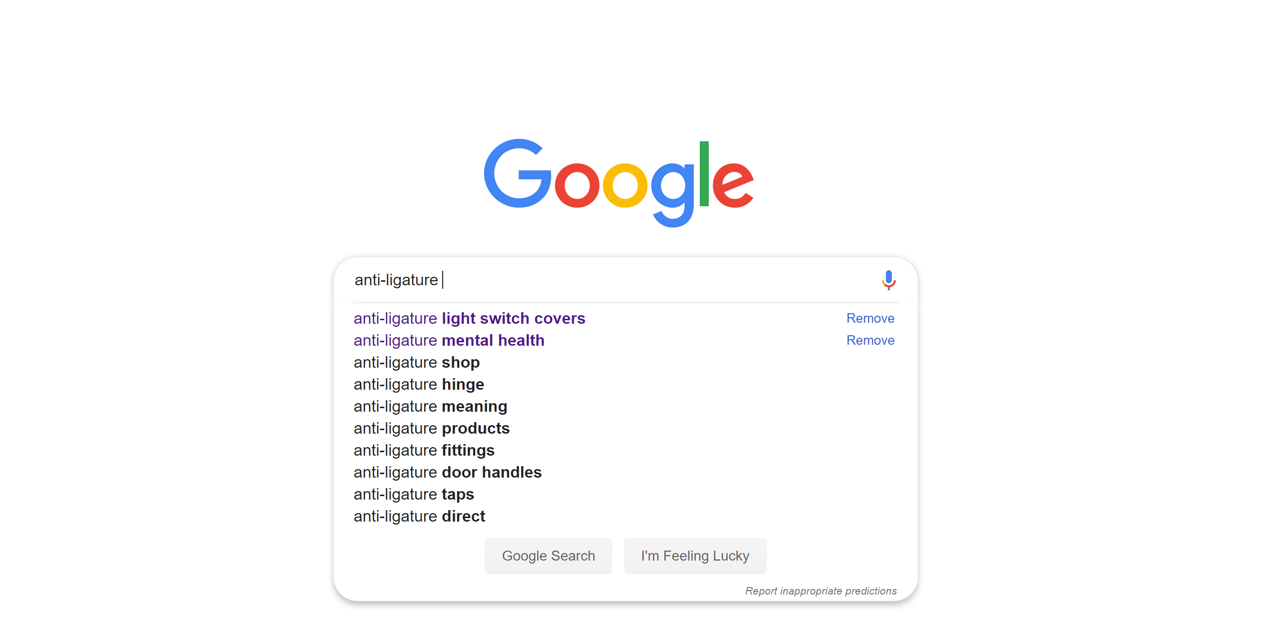This is a detailed screenshot of a Google search page. Dominating the top portion of the page is the iconic, colorful Google logo. Directly below this, within the search bar, the term "anti-ligature" is clearly typed, with a small microphone icon situated on the right side of the bar, indicating the option for voice search. 

Sequential down the list, the search results are prominently displayed and include various entries related to "anti-ligature," such as:

1. Anti-ligature light switch covers
2. Anti-ligature mental health
3. Anti-ligature shop
4. Anti-ligature hinge
5. Anti-ligature meaning
6. Anti-ligature products
7. Anti-ligature fillings
8. Anti-ligature door handles
9. Anti-ligature tape
10. Anti-ligature direct

At the very bottom of the screenshot, two rectangular buttons are visible: one labeled "Google Search," and the other labeled "I'm Feeling Lucky." In the top right corner of the page, the word "remove" appears twice in a small blue font, suggesting additional options or results that can be managed or dismissed.